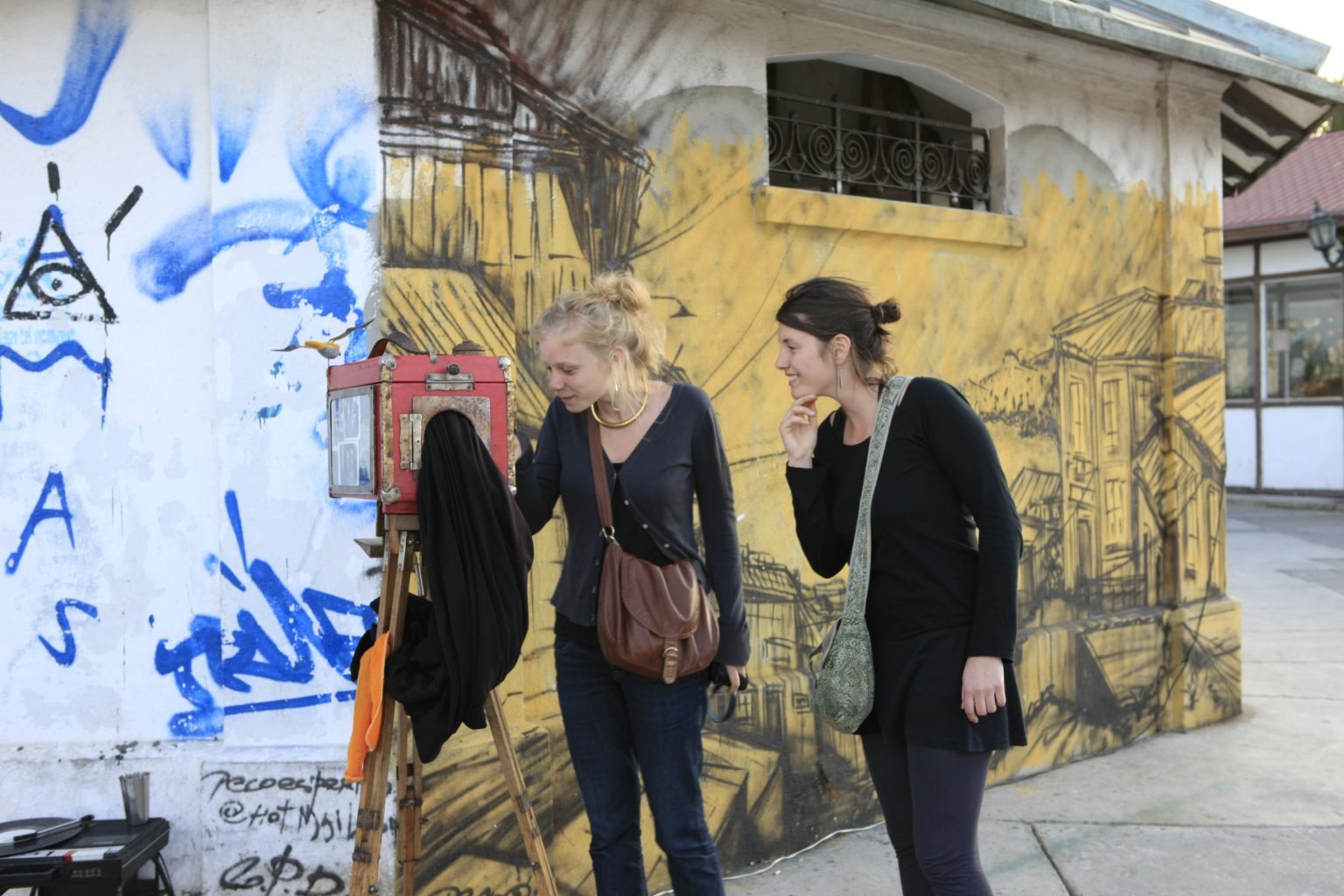The image captures an urban scene featuring two women standing on a clean sidewalk, positioned in front of a rustic, older building adorned with a variety of graffiti, including a prominent pyramid with an eye and numerous names in blue on a white background. The photograph is taken outdoors during the daytime under natural light, suggesting a candid yet possibly staged scene. 

To the right, behind the women, a yellow mural depicting buildings adds a splash of color, executed in a street-art style using pastel or charcoal-like materials. The women are focused intently on a peculiar object: an antique-style camera from the 1800s, identifiable by its red wooden box and a black tarp for the photographer, mounted on a tripod. One woman, a blonde with her hair in a bun, is gently touching the tarp and wears a brown purse along with a prominent golden necklace. The other, a brunette, is dressed casually in a dark long-sleeve shirt, blue jeans, and a jade-colored purse slung around her neck, and she gazes at the camera with a slightly puzzled expression. A sense of curiosity and intrigue emanates from their poses and facial expressions.

In the background, possibly indicative of a tourist-centric location in an older part of the city, another building that looks like a shop or restaurant is partially visible. The overall scene combines elements of urban decay with a hint of historical allure, making it both visually intriguing and rich in narrative detail.